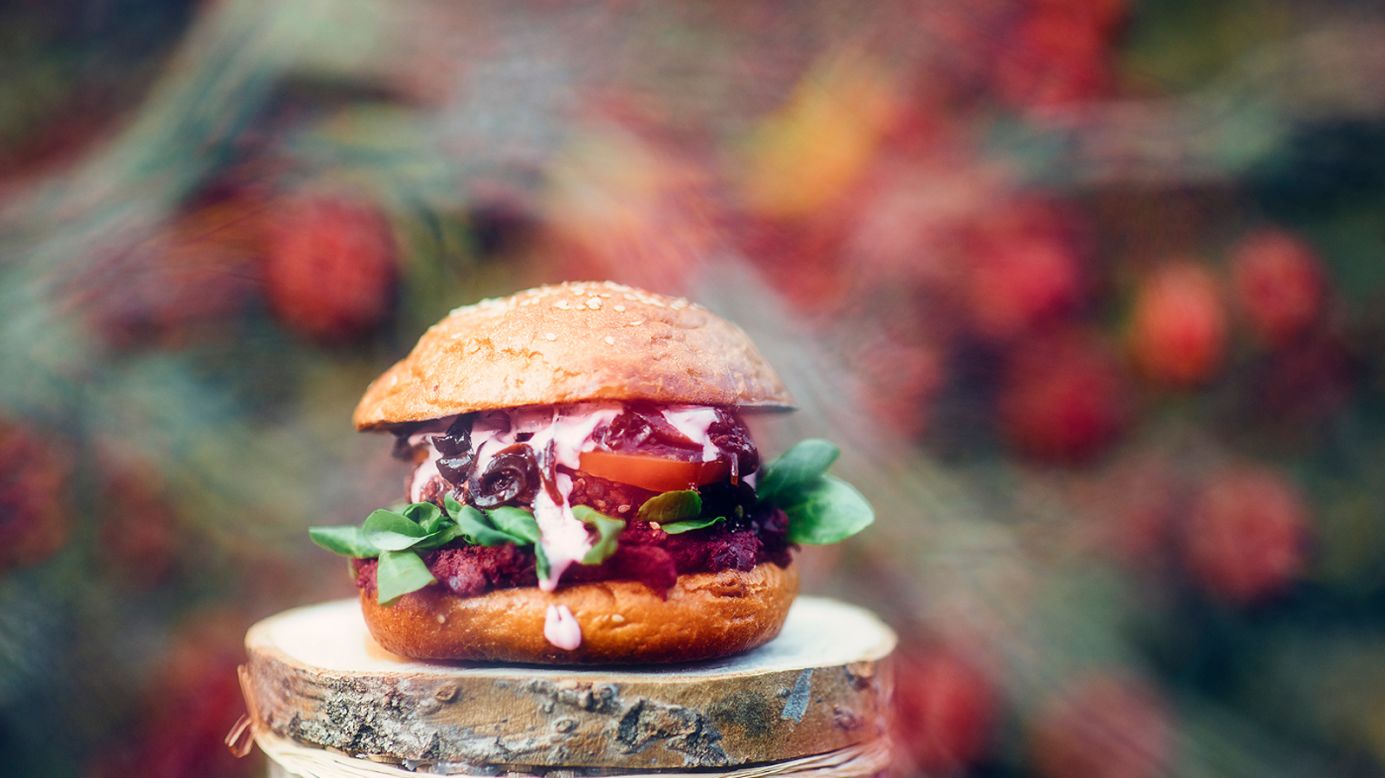The image is a full-color photograph, horizontally oriented without a border, featuring a clearly staged composition. At the front and center is a sandwich, specifically a burger, placed on a circular platform that resembles a tree stump or stone pedestal with a wooden texture. The burger features a toasted, sesame-seeded brioche bun on top and bottom. Sandwiched in between are visible layers of fruit and vegetables, including strawberries, raspberries, tomatoes, green leaves that could be lettuce, and possibly olives. There is also a white sauce, which could be either whipped cream or mayonnaise, oozing from the sides. The background of the image is completely out of focus, creating a bokeh effect. It is filled with colors and shapes, including greens and reds, resembling flowers, apples, or possibly other fruits interspersed with what appear to be swirling white lines like smoke.